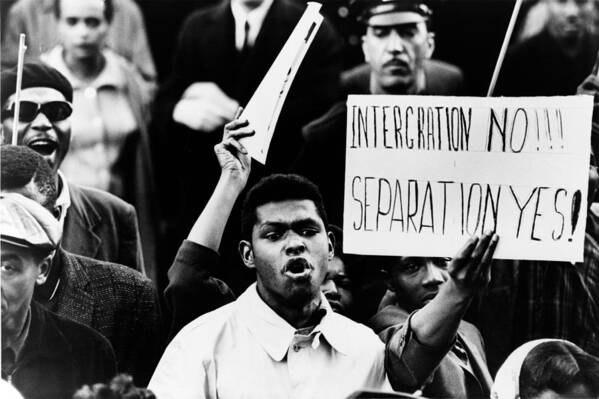In this vintage black-and-white photograph, likely taken during the 1960s to 1980s in the United States, a group of primarily African American men and possibly a few women are participating in a protest or march. The image, captured in an era before color photography was prevalent, exudes a historical atmosphere. The crowd appears energetic, with a mix of people smiling and others yelling or chanting. Prominently, an African American man in the foreground holds a sign that emphatically reads "Integration no!!! Separation yes," suggesting a stance against racial integration, likely due to the pervasive racism of the time. Adding to the scene's intensity, a stern-looking Caucasian policeman, sporting a Germanic-style mustache, stands in the center, heightening the tension and historical context of the photo. The participants are wearing dark or light-colored clothing, typical of the black-and-white photography era, and the overall mood conveyed is one of determined activism amidst a struggle for racial identity and justice.